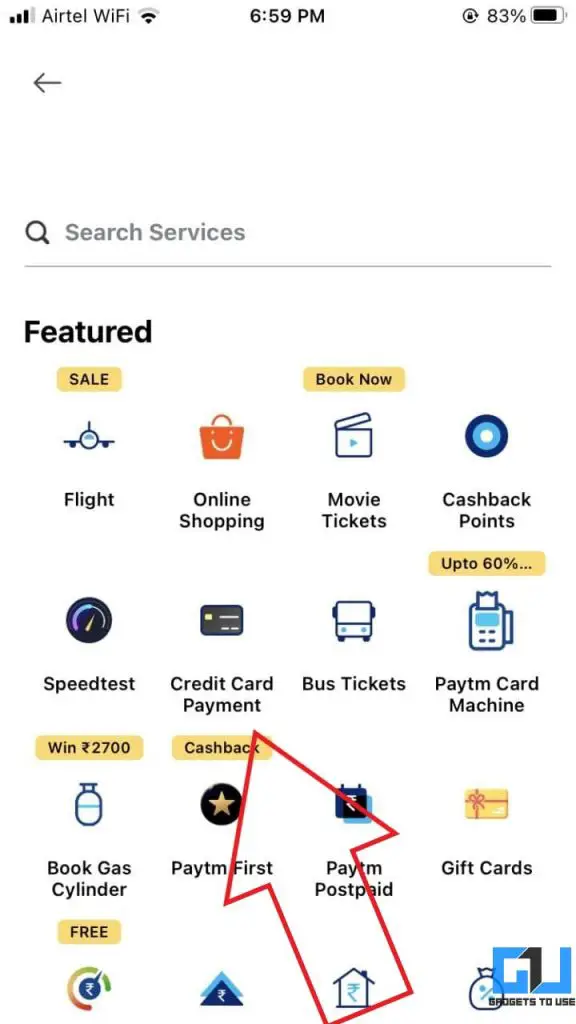This screenshot depicts a detailed interface from a tablet or smartphone. Here's a detailed breakdown of the elements present on the screen:

1. **Top Bar:**
   - **Signal Strength:** Displays three out of four bars indicating the network signal strength.
   - **Wi-Fi Status:** Shows connected to "Airtel Wi-Fi" with two out of three bands active.
   - **Time:** Displays "3:59 PM" prominently in the center.
   - **Security Lock Symbol:** Located on the right, indicating the device is locked.
   - **Battery Life:** Shows 83% battery remaining next to the lock symbol.
   - **Grey Arrow:** Appears on the left side of the top bar.

2. **Main Interface:**
   - **Magnifying Glass Icon:** Black in color, symbolizing a search function.
   - **Search Bar:** Contains grey placeholder text and a grey underline.
   
3. **Features Section:**
   - **Featured Title:** Bold black text labeled "Featured."
   - **Airplane Icon:** Blue and black airplane facing forward with a yellow rectangle above it labeled "Sale" in blue text.
   - **Flight Booking:** Subtext "Blue Light" with an orange shopping bag icon that has white dots and a smiley face, labeled "Order Online Shopping."
   - **Movie Tickets:** Yellow rectangle with an open box showing a cyan play button, a blue border, and white interior, text says "Movie Tickets."
   - **Cashback Offers:** Dark blue circle with layers of cyan and white circles inside, text reads "Cash Out Cashback Points" followed by a rectangle mentioning "Up to 60%."

4. **Other Icons and Offers:**
   - **Speed Test Logo:** Dark blue to purple gradient circle with a cyan and white interior, resembling a speedometer.
   - **Credit Card Payment Offer:** Red arrow pointing to a credit card symbol, followed by "Credit Card Payment" and "Cash Back" within a yellow/gold rectangle.
   - **Bus Tickets:** Icon featuring a silhouette of a bus and text for "PAYTM."
   - **Gas Cylinder Booking:** Cyan blue line and dark blue border resembling a gas cylinder with "Free" written in a gold rectangle.

5. **Additional Features:**
   - **PAYTM First:** Black circle with a golden star and text "PAYTM First."
   - **PAYTM Postcard:** Dark blue tab with white text over a cyan background.
   - **Gift Card:** Gold card with a red bow, labeled "Gift Cards" in white text.
   - **Other Speed Test Type Icon:** Dark blue triangle with a unrecognized denomination, partially cut off.

6. **Miscellaneous:**
   - **House Icon:** Cyan blue with similar styling as the speed test icon, partially cut off.
   - **Discount Bag:** Illustrates a bag with a percentage sign.
   - **Gadgets in Use:** Large blue square with two 3D white squares having noticeable shadows, labeled "Gadgets to Use."

This detailed narrative captures the various elements and information displayed on the screen.